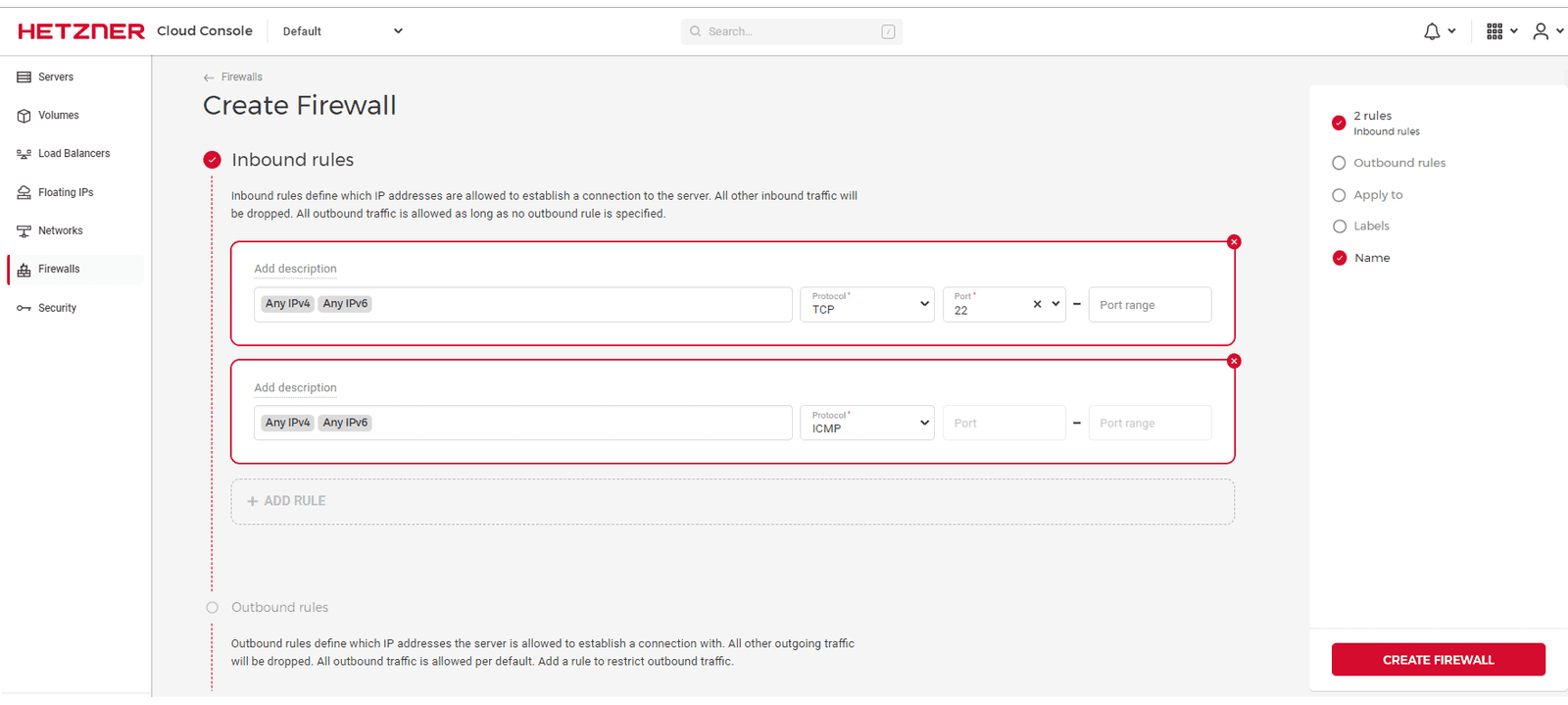The image showcases a structured interface with multiple elements. 

At the very top, a thin gray line runs horizontally, beneath which "H-E-T-Z-N-E-R" is prominently displayed in bold red text. To the right of this text, some smaller, indistinguishable words are present. Below this header, there is a light gray search bar with a magnifying glass icon within it, accompanied by a word next to the icon. Towards the right-hand side, icons for notifications, settings, and user account actions are visible, though some details are too small to discern clearly.

On the left-hand side, there are several symbols each followed by text. These include a total of six symbols each paired with corresponding text, the last of which is marked by an adjacent red line followed by more text beneath it. Further down, a gray button labeled "Create Firewall" is visible, followed by a red circle and a vertical red line extending downwards next to the label "Inbound Rules." Below this, there is text which is too small to read.

The interface also includes various actionable areas outlined in red and gray. A rectangle outlined in red with a red dot on its upper right-hand corner contains unreadable text. Similar rectangles, this time outlined in gray, appear below; the number is difficult to confirm but it appears there are four. Another red-outlined rectangle with a red dot on the top right also appears, with further text and more gray-outlined rectangles beneath it. One of these gray-outlined rectangles has some illegible words beneath it.

On the extreme right, there is a white button, a red circle with text next to it, and a series of gray-outlined circles, each accompanied by its own text. Another red circle with text is also seen on this side of the interface. At the bottom of the image, a red button with more illegible text can be found.

In summary, the image presents a structured interface with a header, search bar, various icons, labeled symbols, action buttons, and several outlined rectangles featuring either red or gray accents.